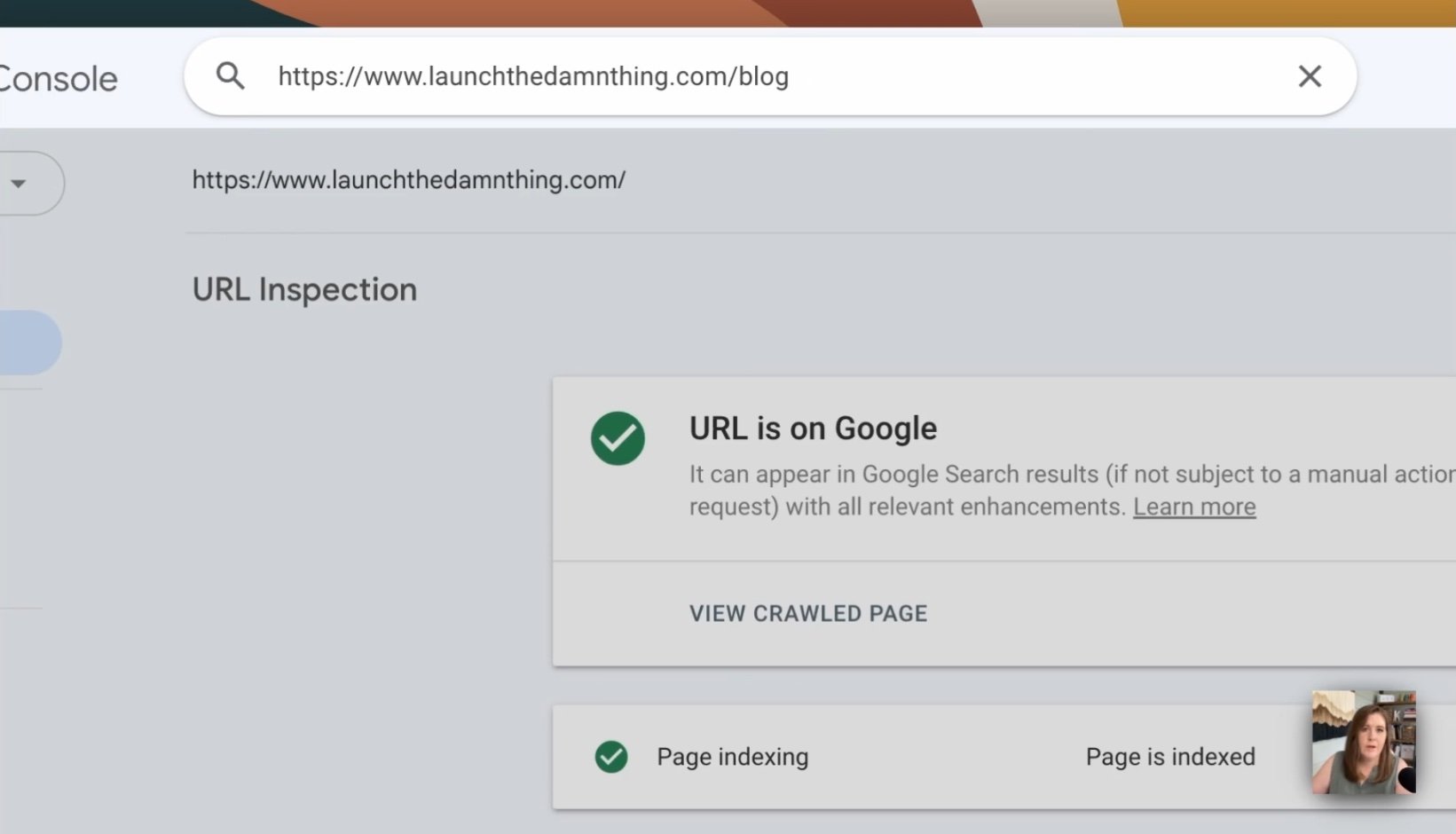The image captures a screenshot of a website viewed within a browser. At the top center, the URL bar displays "https://www.launchthedamnthing.com/blog," accompanied by a magnifying glass icon on the left and an "X" on the right. In the top left corner of the browser window, the word "Console" is visible. Beneath the URL bar, the website's name, "https://www.launchthedamnthing.com," is displayed again alongside a small down arrow.

Dominating the central portion of the image is the heading "URL inspection." Below it lies an empty space, followed by a section in the bottom right featuring two distinct boxes. The upper, larger box states "URL is on Google," highlighted by a green circle containing a white check mark. The accompanying text reads, "It can appear in Google search results if not subject to a manual action request. With all relevant enhancements, learn more," with "learn more" underlined for emphasis. Beneath this, the second box is labeled "Page indexing."